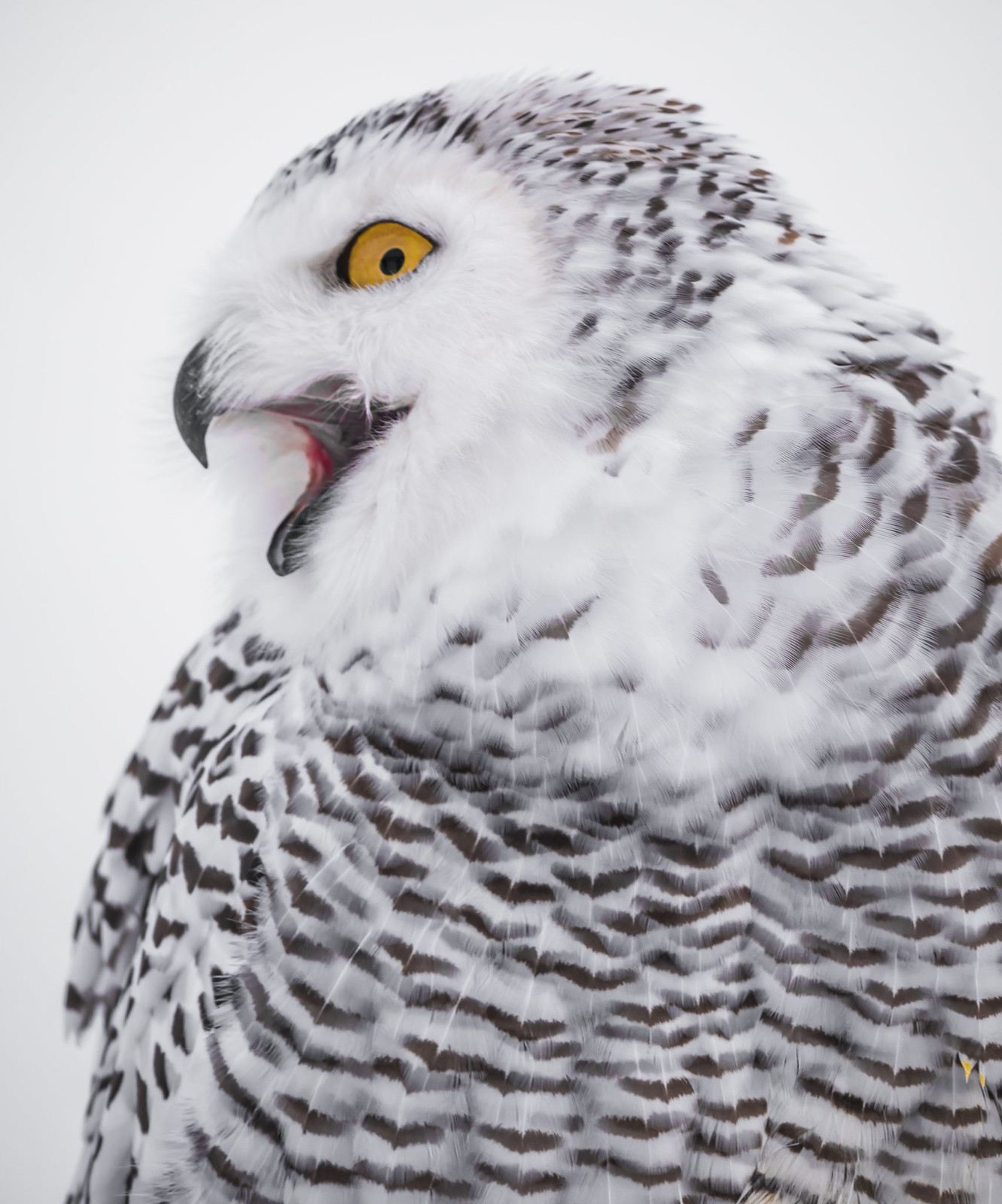The image features a striking close-up of a snowy owl with predominantly white plumage marked by numerous gray spots at the tips of its feathers. The owl's face is pure white, dominated by intense yellow eyes with black pupils and a hooked, black beak, which is currently open, revealing the pink interior of its mouth as if caught mid-yawn or mid-call. The owl is gazing intently towards the top left corner of the image, giving an impression of focus or alertness. The composition cuts off much of the owl’s lower and right side, leaving its feet, claws, talons, and much of its body unseen. The background is a featureless expanse of gray, creating a stark contrast that further highlights the owl's striking features.